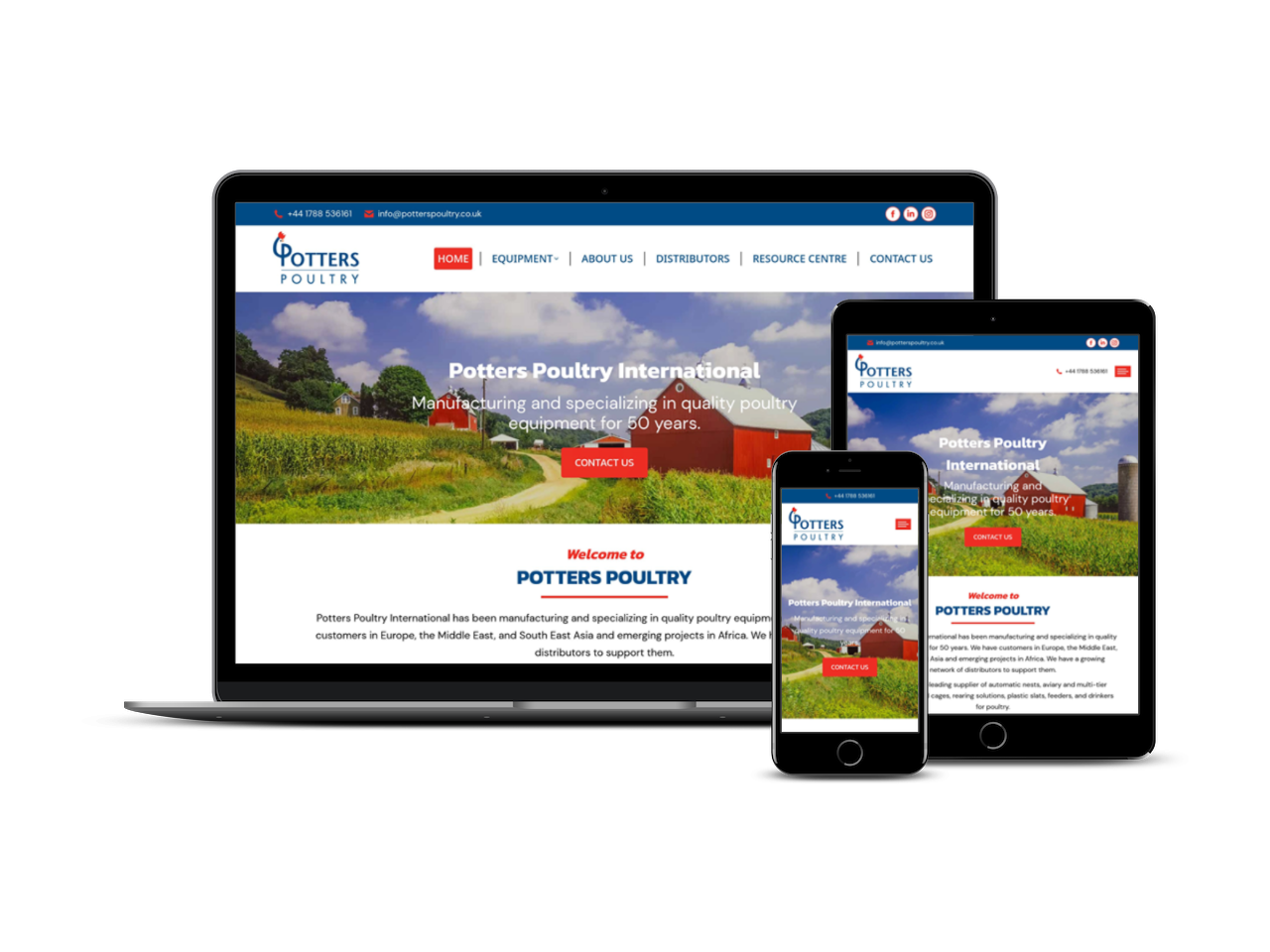The photo showcases three electronic devices prominently displaying the same webpage for Potter's Poultry. Dominating the image is a laptop, centered and occupying most of the frame. To its right, slightly overlapping about two inches of the laptop's side, is a tablet. A smartphone partially overlaps the left inch of the tablet and covers about an inch of the bottom right section of the laptop.

All three devices clearly show the Potter's Poultry website, each providing a slightly altered view due to their differing screen sizes. The laptop screen displays a white banner at the top, accompanied by an image of a farmstead, and informational text at the bottom. The tablet mirrors this layout albeit on a smaller scale. The smartphone screen shows the Potter's Poultry title, a picture of the farmstead, and a condensed view of the content.

The website menu visible on all screens includes options like Home, Equipment, About Us, Distributors, Resource Center, Contact Us, and highlights Potter's Poultry International—a company specializing in manufacturing quality poultry equipment for 50 years. A "Contact Us" button and a welcome message are also visible, though partially cut off: "Welcome to Potter's Poultry. Potter's Poultry International has been manufacturing..." The interfaces also show social media icons for Facebook and Instagram at the top, suggesting ways to connect with the brand.

In sum, the image emphasizes the consistency of the Potter's Poultry website across different devices, showcasing its adaptability and user-friendly design.